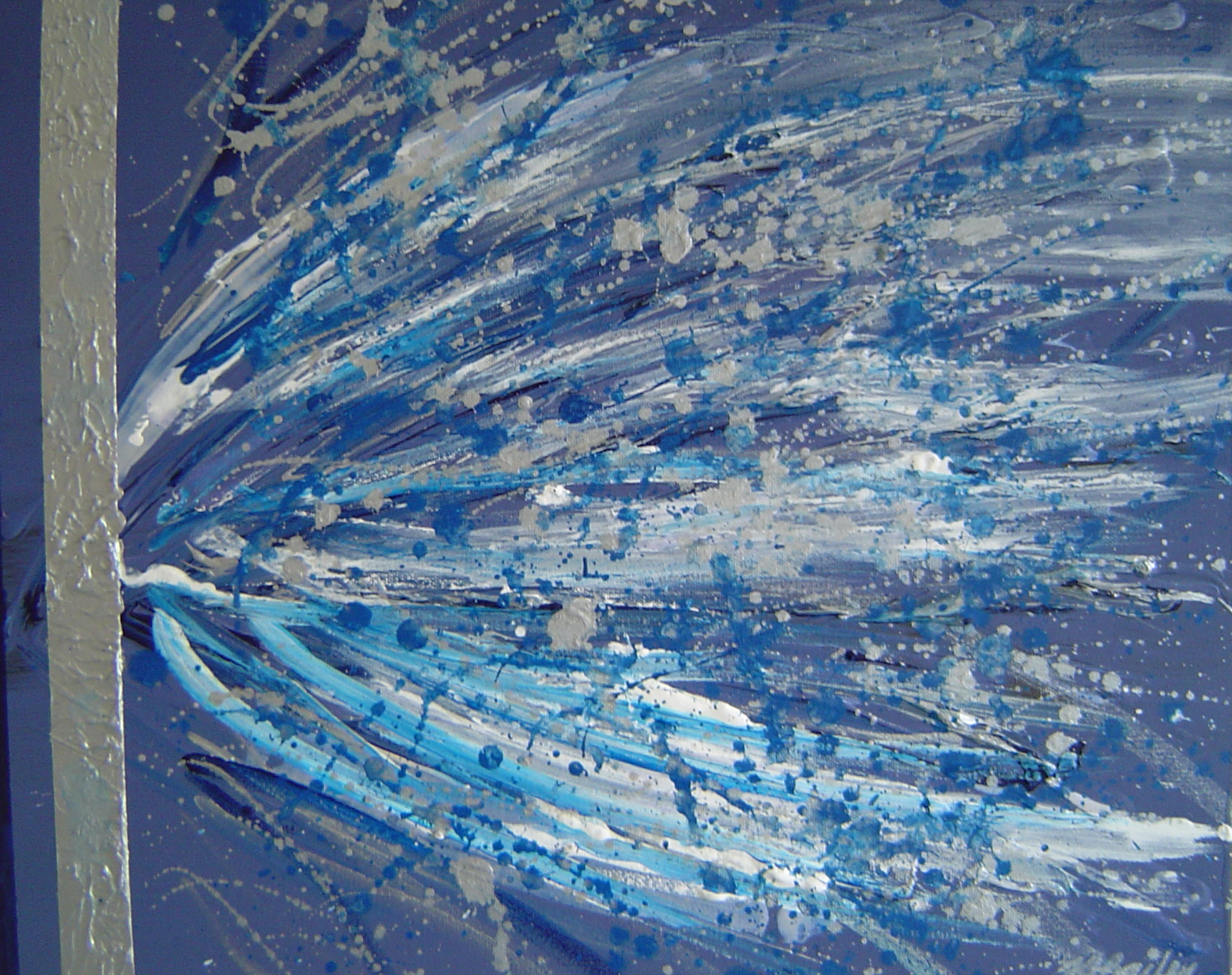This is an image of an abstract painting set against a dark blue background. Dominating the left side is a very thin, textured vertical line in gray, which extends from the top to the bottom of the painting. From this vertical line, brush strokes fan out horizontally, creating a dynamic impression of movement similar to fireworks at night. These brush strokes, mixed with colors including dark blue, sky blue, gray, and white, vary in intensity; the topmost strokes are more gray with blue hints, the middle section incorporates more white, and the bottom strokes blend more blue and white. In addition to these brush strokes, splatters of white, light blue, dark blue, and black overlay this composition, adding depth and texture to the overall artwork.